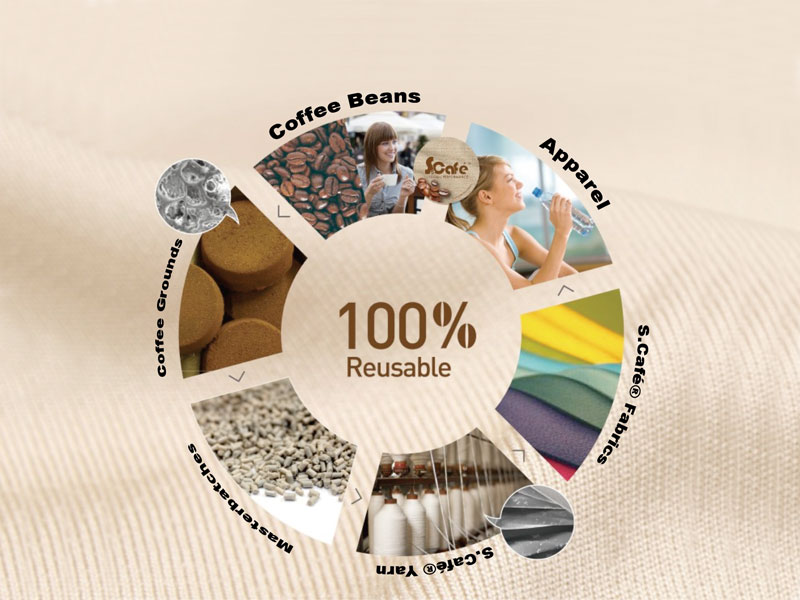The image is a detailed advertisement featuring a beige fabric background, resembling a knit cloth or sweater, which is slightly curved and blurred in some areas for effect. At the center of the image, in dark brown text, are the words "100% reusable." Surrounding this central text is a circular arrangement of six images, each within an arc-shaped frame, accompanied by black captions describing different uses of a brand's products. 

Starting from the top and moving clockwise: 

1. **Coffee Beans**: A photograph of coffee beans and a woman holding a coffee cup.
2. **Apparel**: A woman holding a water bottle, illustrative of reusable apparel.
3. **Escafe Fabrics**: Multicolored fabrics, including green, yellow, blue, and purple.
4. **Escafe Yarn**: Spindles of yarn depicted in various colors.
5. **Master Batches**: An unclear image relating to the term, possibly referring to raw material processing.
6. **Coffee Grounds**: Coffee disks shown alongside ground coffee.

The design emphasizes reusability and sustainability across various products, visually organized in a circular fashion around the central message.